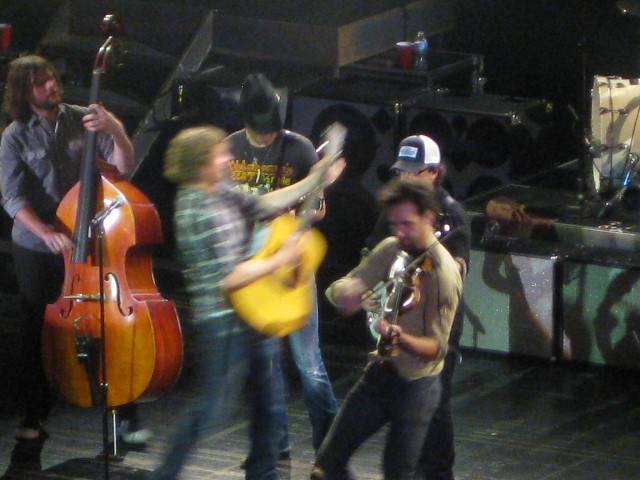This is a color photograph captured indoors during a concert or rehearsal. The image is dominated by a dark background and features five musicians in the spotlight, primarily positioned towards the left and center of the frame. On the far left, there is a tall man with long brown hair and a beard, wearing a blue shirt and playing a large, browny-orange bass fiddle or cello. Moving right, a blurred individual with blonde hair, a blue striped shirt, and blue jeans is seen playing a yellow guitar. Just behind this musician is a person in a black cowboy hat and a black t-shirt featuring a red, yellow, and green logo. Towards the center-right, another musician with a goatee, brown hair, green shirt, and black jeans is playing a fiddle or small violin, facing the camera directly. Behind him stands a figure wearing a black and white baseball cap, possibly playing a banjo. The stage features dark, almost puke-brown steps without hand railings on the left, leading up to the wooden, dark-colored floor. Various old-style speakers with silver fronts and fake wood tops flank the setup, casting shadows onto a barrier behind the musicians. The overall scene is characterized by motion blur, likely indicating the band's energetic performance amidst the dimly lit environment.